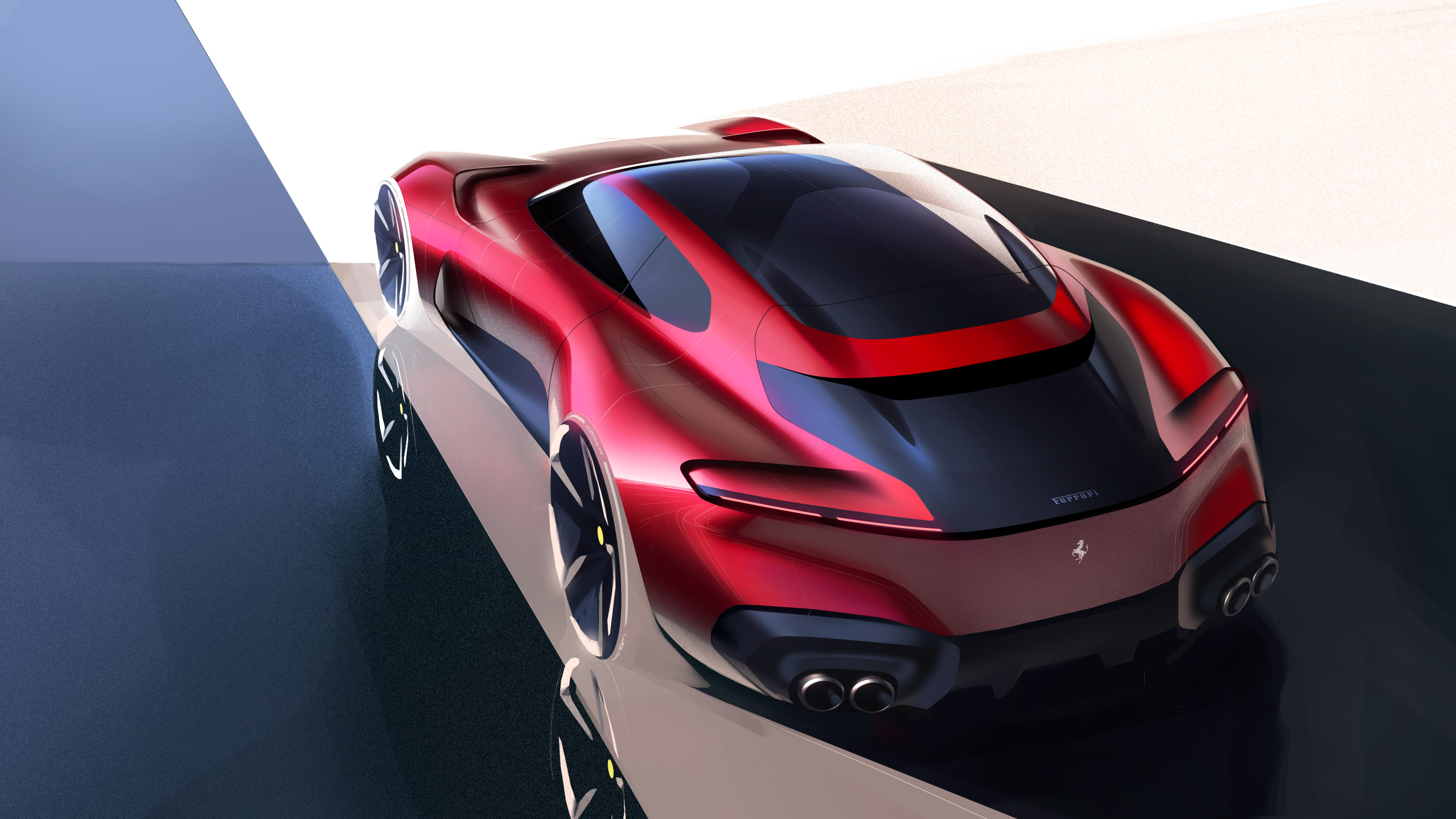The image depicts a hyper-realistic rendering of a high-end luxury sports car, most likely a Ferrari. The car boasts a sleek, modern design and is predominantly red with a distinctive black panel on the trunk area. It features a large sunroof that replaces the traditional roof and has two prominent exhaust pipes on either side of its rear. The car is angled away from the viewer, showcasing its back and left side. It rests on a platform with a black and dark blue floor, with elements of the background including white, blue, and tan sections. The Ferrari logo is visibly prominent on both the front and back of the car, highlighting its esteemed brand identity. The overall image exudes a shiny, polished finish, emphasizing the vehicle's sporty and luxurious appeal.